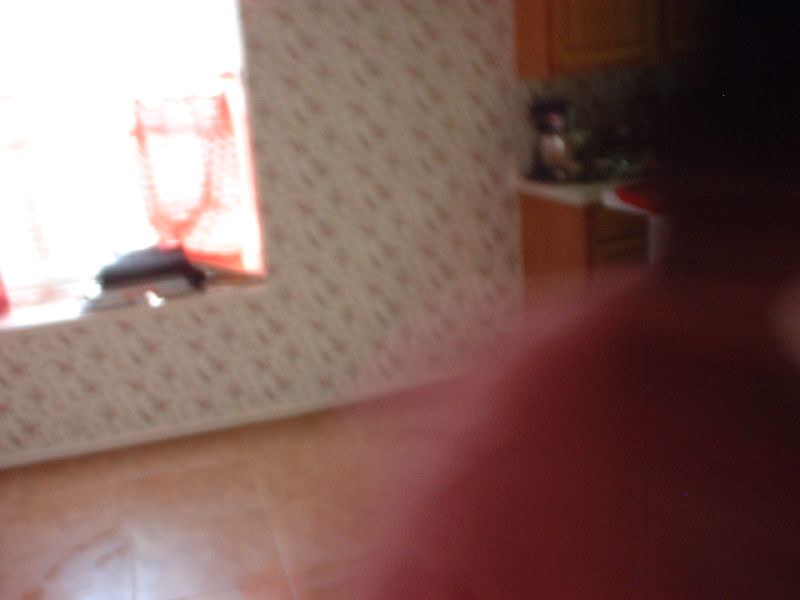A blurry interior shot of a home taken at an angle, depicting an orangish tile floor and a wall with a window on the left. Sunlight streams in through the window, casting light on an assortment of unidentifiable items on the windowsill. To the far right, a cupboard and a countertop are visible, with indeterminate objects resting on the counter. In the foreground, occupying the bottom-right corner, is the indistinct form of a person wearing a pinkish top, likely the back of their head and shoulder. The photograph appears to have been captured without adequate lighting and with movement, contributing to the overall blur.